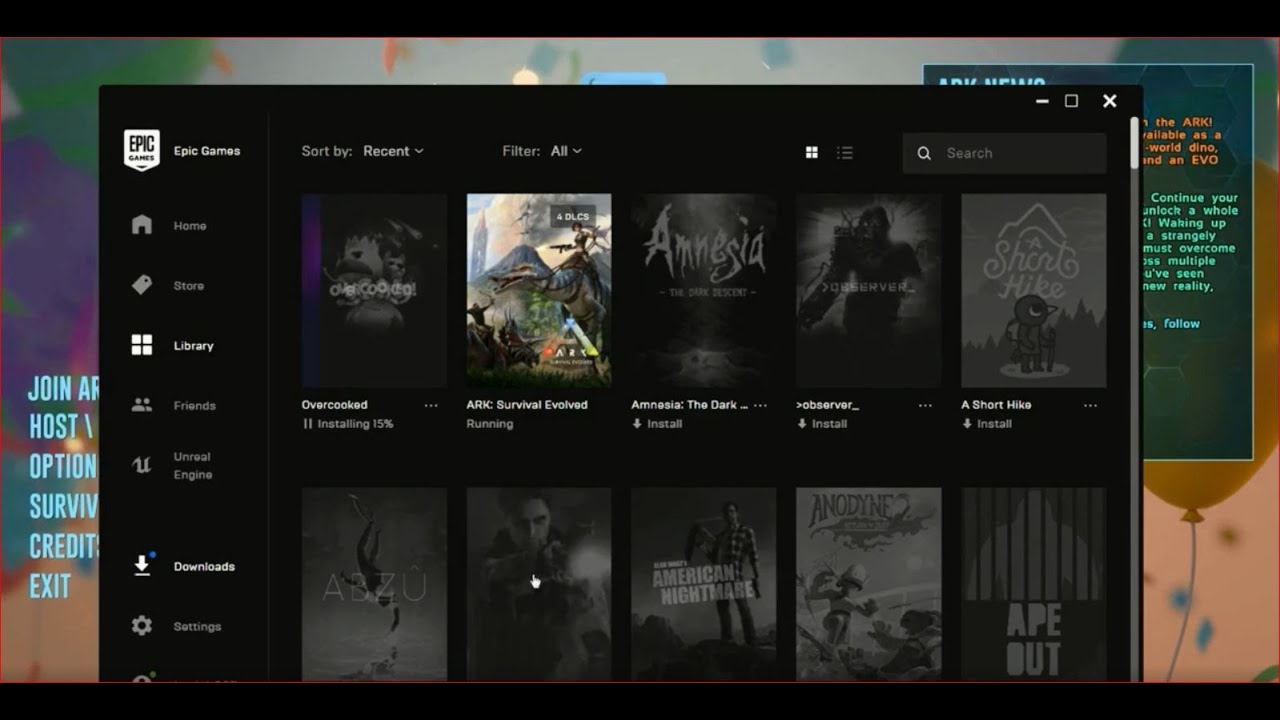The image depicts a web page from a browser window superimposed on the background screen of a computer. On the left-hand side of the interface, there is a navigation menu with options labeled: Epic Games, Home, Store, Library, Friends, Unreal Engine, Downloads, and Settings. The top bar of the webpage features filters with options to "Sort by Recent" and "Filter All," along with toggles for displaying content as a grid or a list.

In the main content area, a list of games is displayed. At the top of the list is "Overcooked," which is currently 15% installed. Following that, "Ark Survival Evolved" is indicated as running. "Amnesia," "Observer," and "A Short Hike" are shown with options to install. The next row of games includes "Abzu," "American Nightmare," and "Ape Out," but their installation or running statuses are not visible in the image.